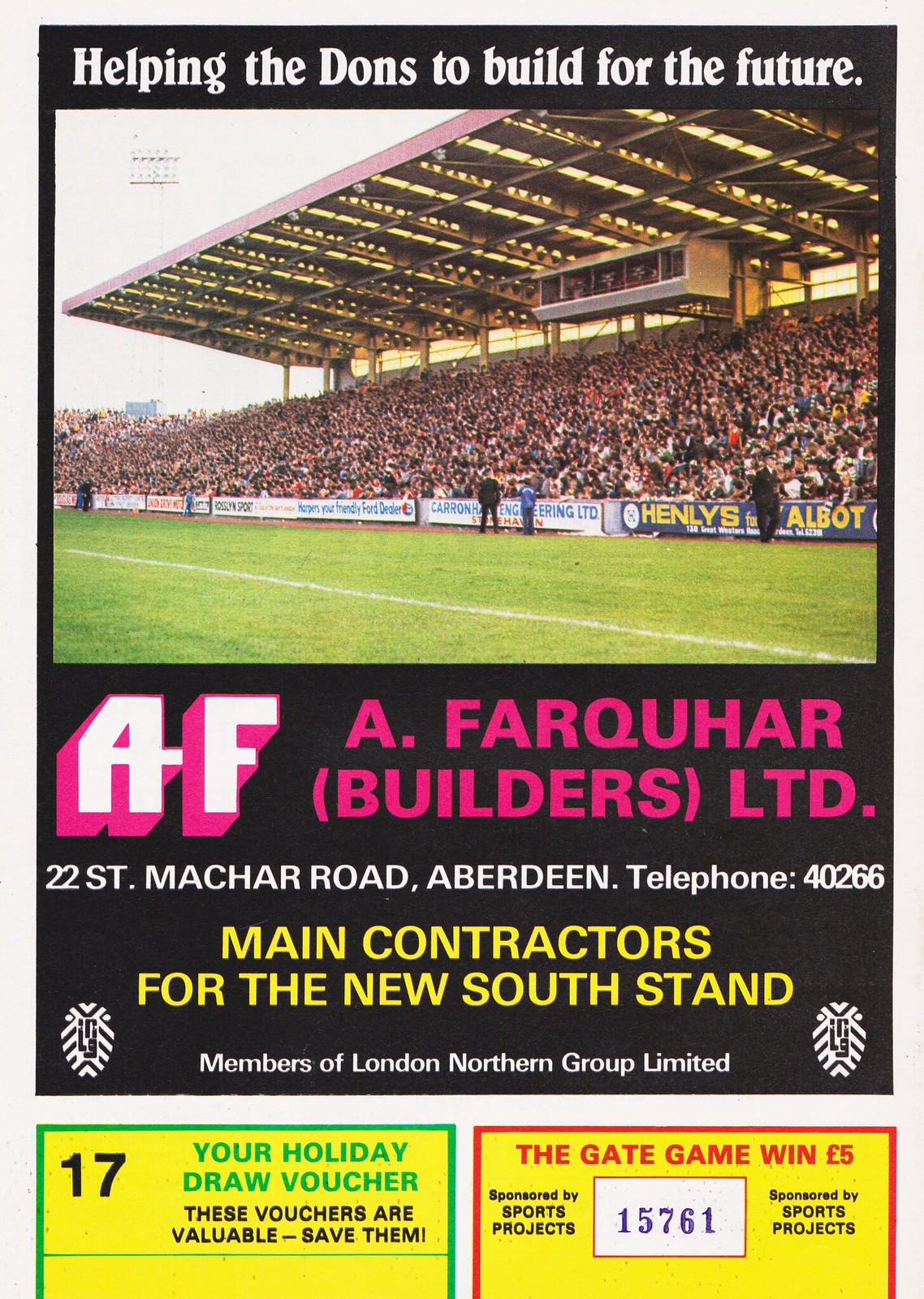The image appears to be the cover of an old match day program or flyer with an aged white background. At the top, inside a large black rectangular box, it reads in white text, "Helping the Dons to build for the future." Below this is an image of a large football stadium, showcasing a grass field at the center. The spectator area is prominently displayed, featuring a huge roof and filled with a sizable audience. In the middle of the image, within another black section, it says "A. Farquhar Builders Ltd." in white and pink text. Following that, in white text, it provides the address: "22 St. Machar Road, Aberdeen, Telephone 4266." In yellow text, it is noted that they are the main contractors for the New South Stand and members of the London Northern Group Limited. At the bottom, there are two distinctive yellow rectangles. The first states, "Your holiday draw voucher. These vouchers are valuable, save them," and displays the number 17 with a green outline. The second rectangle states, "The gate game win five pounds, sponsored by Sports Projects," with a red outline.